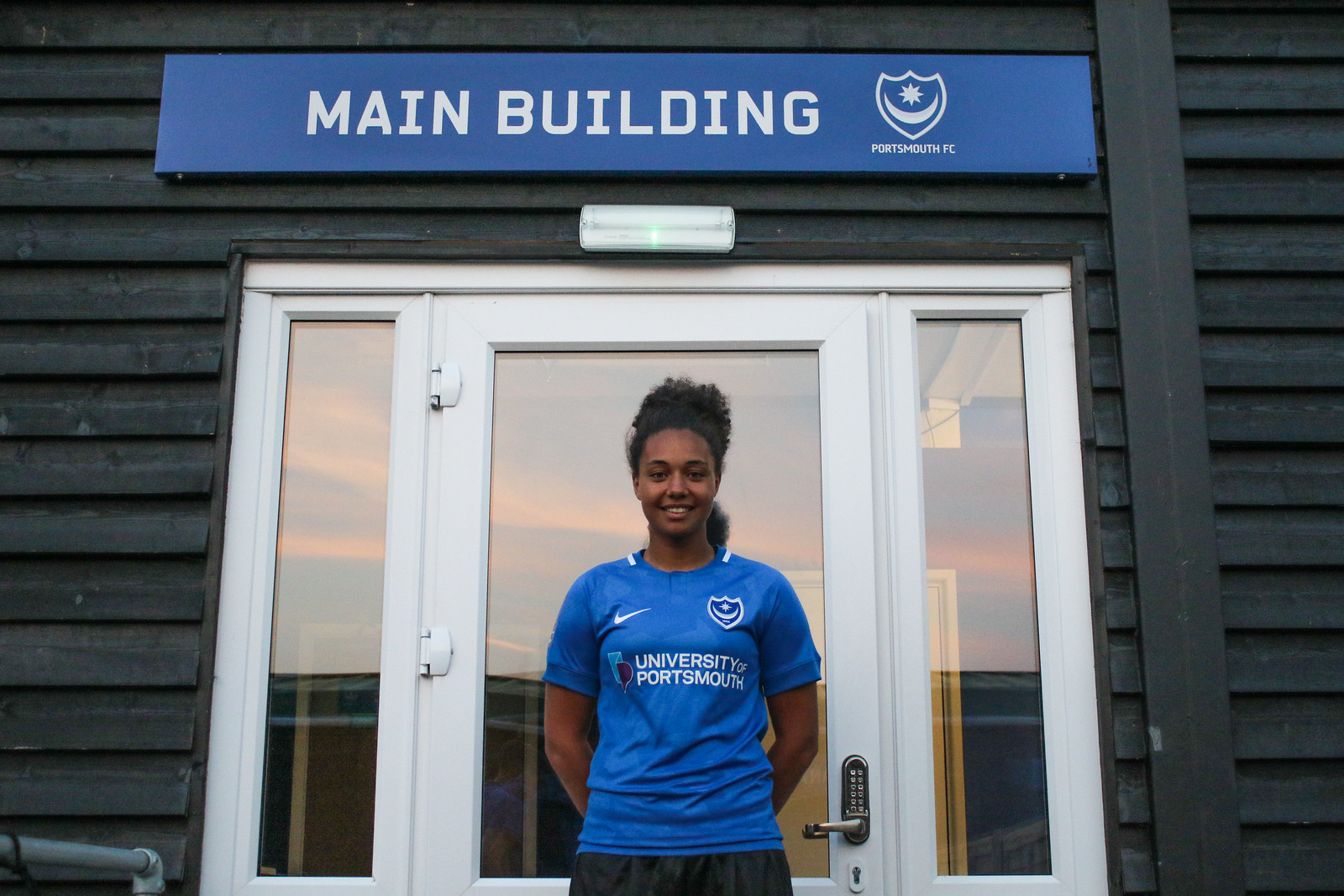In this photograph, taken during the daytime, a young black woman stands outside in front of a distinctive building. She has a brown complexion and her black hair is styled in a high ponytail, which poofs slightly. She wears a blue short-sleeve shirt detailed with the Nike logo and a shield, bearing the text "University of Portsmouth" in white lettering. She pairs this with black shorts. The woman is smiling directly at the camera with her arms positioned behind her back, and the photo captures her from the upper thigh up.

The building behind her is characterized by horizontal, very dark gray wood siding. Above the glass entry door, which is framed in white metal and flanked by two smaller glass panels, there is a rectangular blue sign with white lettering that reads "Main Building." Just below this sign is a small rectangular white light. The door lock is notable for having a numbered keypad for security. The building is identified with symbols and text associated with the University of Portsmouth, contributing to the academic and official atmosphere of the setting.